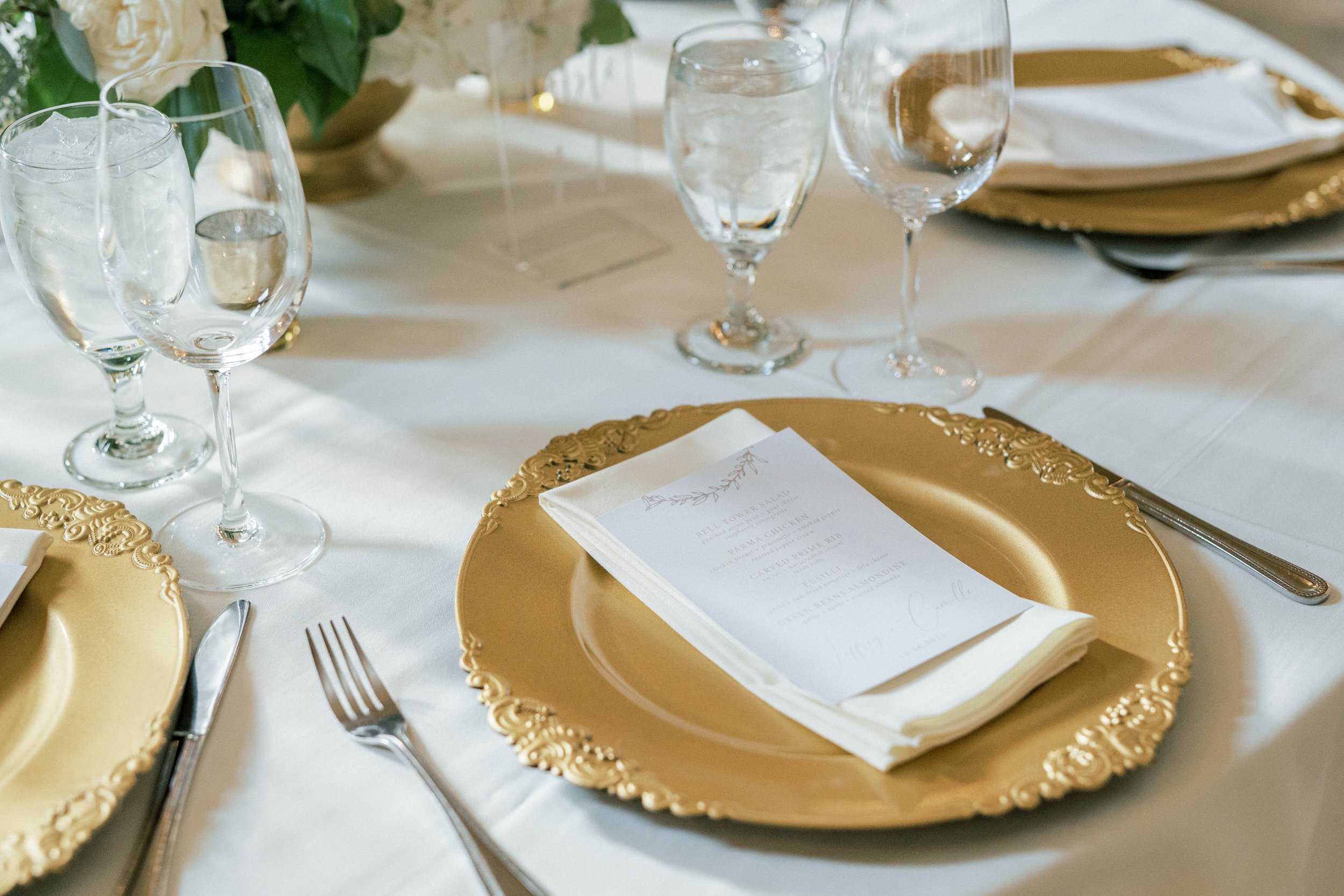In this elegant photograph of a finely set dinner table, the focus is on a central place setting surrounded by other identical settings, all on a pristine white tablecloth. The plates are adorned with a rich gold color featuring intricate garland-like decorations on all four sides, giving a regal and sophisticated appearance. A folded white napkin, possibly linen, rests in the center of each plate, with a piece of white paper containing dark text placed atop the napkin. Flanking each plate are a silver fork on the left and a silver knife on the right. The background showcases an empty wine glass and a goblet filled with ice water, arranged consistently across the table.

In the middle of the table, a brass pot holds a beautiful arrangement of white roses and green leaves, adding a touch of natural elegance. The entire scene is bathed in a soft, soothing light, enhancing the table’s refined ambiance. The photograph is slightly longer in width than height, capturing the top right corner where the floor appears grayed out. Apart from this, small plastic place markers are visible in the background, indicating the seating arrangement. This image perfectly captures the sophisticated and inviting atmosphere of a formal dinner setting.